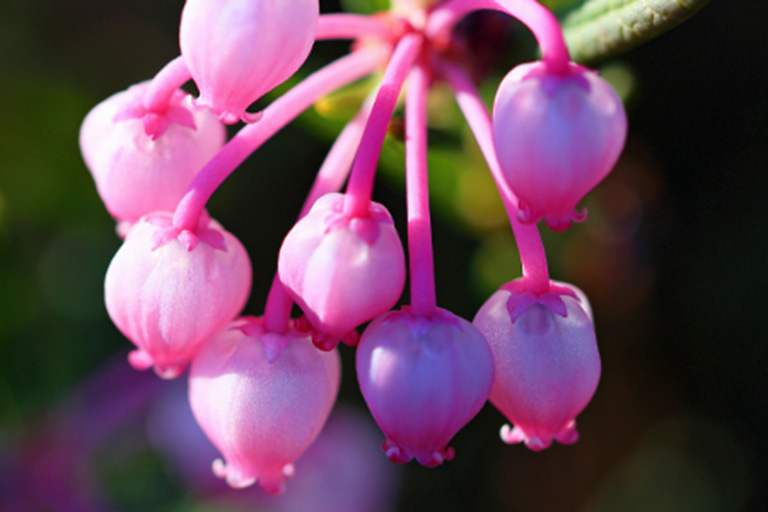This richly colored outdoor photograph captures an up-close, landscape-oriented view of a vibrant cluster of flowers hanging gracefully from a vine. The main subject is a group of eight tiny, bulbous flowers, each delicately drooping downward due to their own weight. The flowers exhibit a light neon-pink hue with subtle purple undertones, giving them a lively and vibrant appearance. Their rounded shapes with ruffled bottoms are reminiscent of little closed pitcher shapes or cotton balls. The background, a smoothly blurred mix of greens, pinks, yellows, and oranges, serves to intensify the prominence and vivid color of the flowers, making them the striking focal point of this stunning floral portrait.